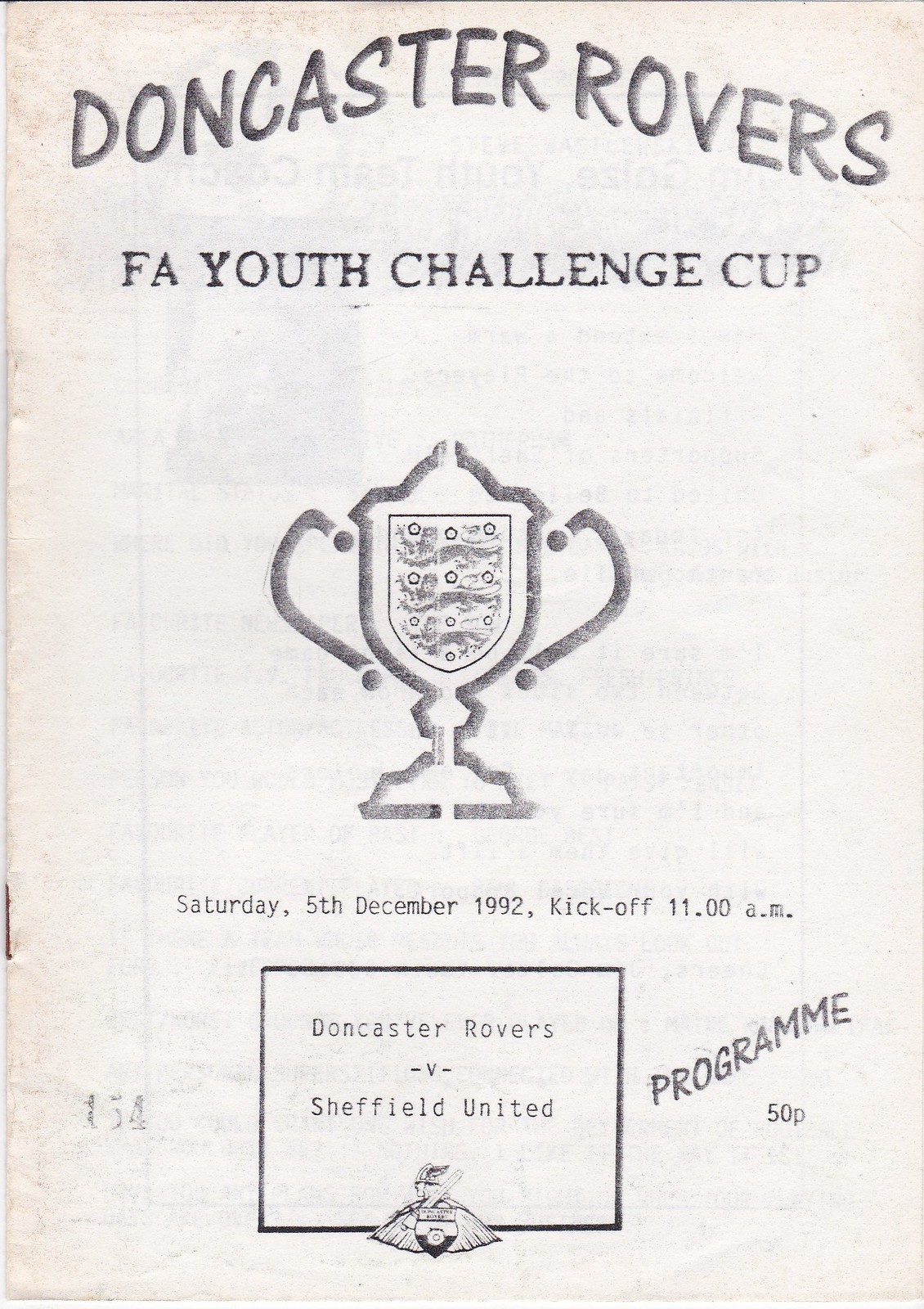The image depicts a weathered, off-white page from an old soccer program booklet. At the top, in a curving, marker-like font, it prominently reads "Doncaster Rovers." Beneath this header, in all capital letters, it states "FA Youth Challenge Cup." Below this text, there's an illustration of a trophy cup with two large handles. The trophy has a shield in the middle adorned with stars. Continuing down the page, the information reads: "Saturday 5th December 1992, kickoff 11 a.m." This is followed by "Doncaster Rovers versus Sheffield United" located within a small rectangle. To the left of this rectangle, the number "154" is faintly visible, while on the right side, it says "Program 50p." Additional details include a rusty staple on the left side of the booklet, indicative of its age, with some ink bleed visible from the other pages, though not enough to read. Near the bottom, there is an illustration of a soldier with a winged helmet, holding a sword, and with a shield and cape, adding a decorative element to the program.